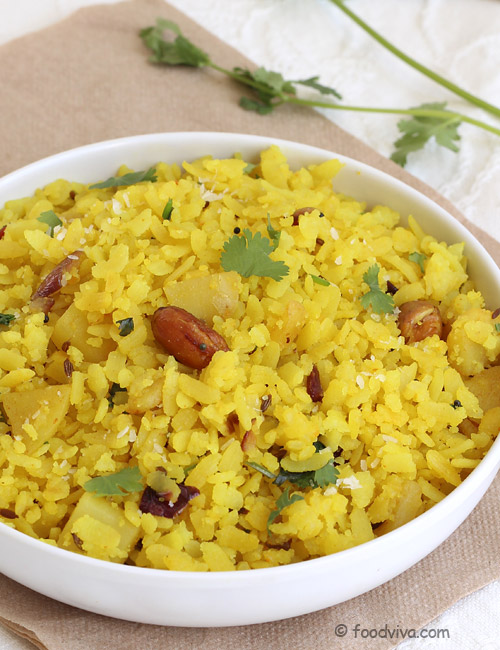The image depicts a white bowl filled with vibrant yellow rice, adorned with scattered cilantro leaves and brown beans. The dish also appears to contain small pieces of potatoes or possibly peanuts. The bowl is set on a light brown napkin, which rests atop a white tablecloth. In the background, a sprig of cilantro can be seen. Additionally, there is a black text watermark on the lower right corner of the image that reads "foodviva.com." The overall presentation suggests a delicious and intriguing meal.